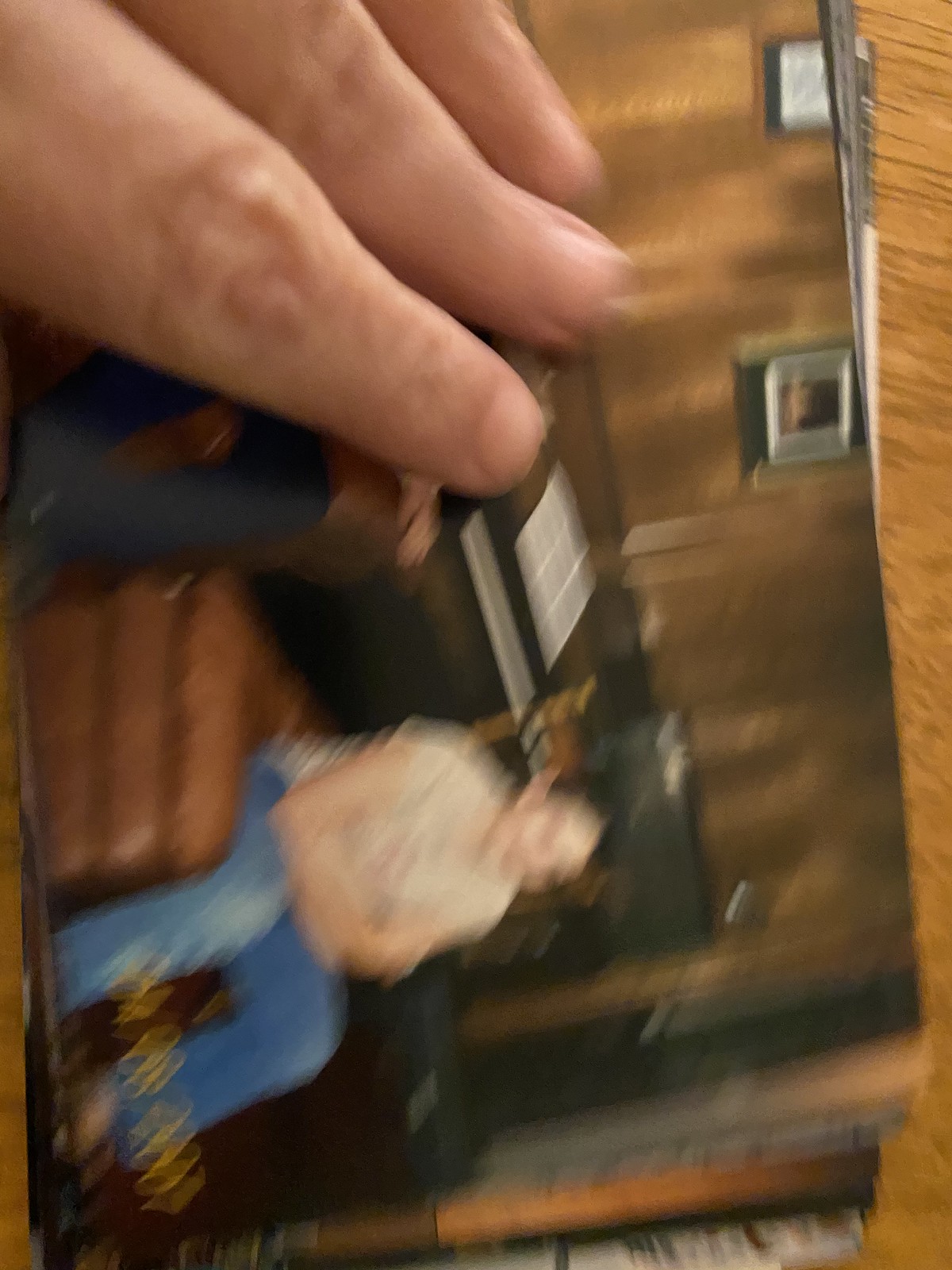The image depicts a printed photograph of a person seated on a leather ottoman, with a piano or organ visible in the background, suggesting an indoor setting. The photo appears to be part of a larger stack, oriented sideways. A male Caucasian hand, showing three fingers, is grasping the top of the image, adding a personal touch. The photograph itself is quite blurry, with a visible date stamp indicating April 8, 2007. The room in the photograph features predominantly brown tones, including brown paneling on the walls, enhancing the vintage, homey atmosphere.